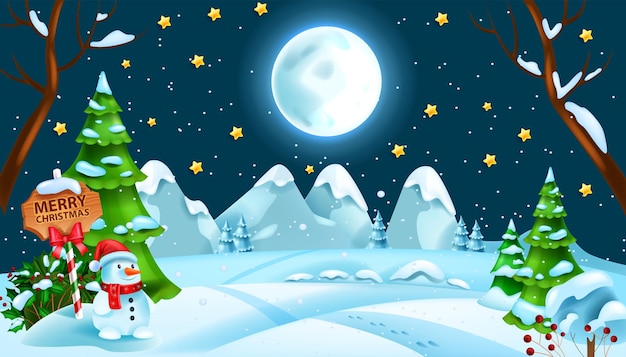This image is a vibrant, cartoonish illustration reminiscent of a Christmas card, depicting a cheerful winter wonderland. The night sky is a deep, dark blue, adorned with a bright, full moon casting a silvery glow, yellow stars, and white dots suggesting twinkling heavenly bodies. The ground is blanketed in heavy snow, with a light dusting still falling, creating a magical, wintry atmosphere.

Dominating the scene is a jovial snowman situated on the bottom left. He wears a red Santa hat with white trim, a matching red scarf, has a classic carrot nose, two black eyes, and three buttons down his front. He stands beside a striped signpost resembling a candy cane, embellished with a red bow, reading "Merry Christmas." The sign itself, capped with snow, adds a festive touch.

In front of the snowman is a tall, green Christmas tree dusted with snow. Surrounding the scene are branches, some barren and snow-laden, while others, likely spruces, stand robust with their snowy coverings. There are also vibrant green holly leaves with clusters of red berries completing the festive scenery. In the background, there are snowy mountains or hills, enhancing the depth and wintry essence of this endearing holiday illustration. 

Overall, the image is a delightful representation of a snowy, festive Christmas night, perfect for a child's holiday illustration or a heartwarming Christmas card.